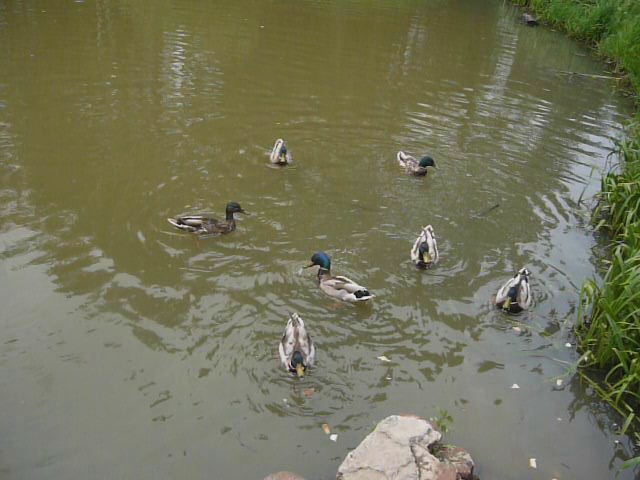This photo captures a murky, outdoor pond with a greenish-brown hue. The pond is still and shows signs of pollution or food debris, with pieces of bread seen floating, suggesting the ducks are feeding. There are seven ducks, resembling mallard ducks, with iridescent green heads and brown and white feathered bodies marked by distinct black stripes. Their beaks are a green-yellow color. The ducks are dispersed across the pond, each appearing to be searching for food with their heads pointed downwards. In the foreground, there is a large rock, and along the right edge of the pond, the grassy bank is visible.